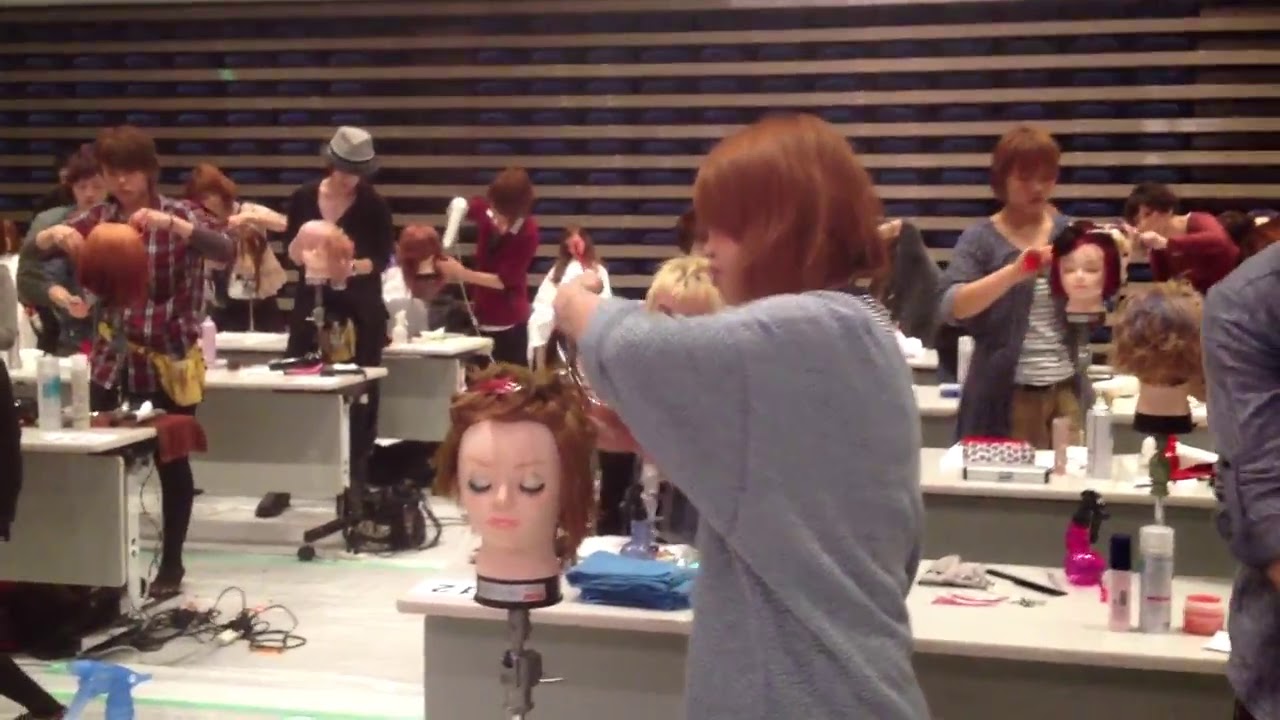The image depicts a bustling classroom filled with beauty students, primarily women of Asian descent, actively engaging with mannequin heads to practice various hairdressing techniques. These learners are situated at several desks aligned in rows throughout the room. Each desk is cluttered with hair products, sprays, scissors, combs, and other beauty equipment. The women appear to be performing a range of tasks, including cutting, dyeing, and shampooing the mannequins' hair, most of which is depicted as a reddish hue. 

The classroom features a wooden, white floor and a backdrop with parallel wooden stripes against a black surface. In the foreground, a young woman with red hair, wearing a gray t-shirt, focuses intently on treating a red-haired mannequin head. Her desk is similarly laden with various hairdressing tools. An assortment of cables and electrical equipment can be seen on the floor in the bottom left corner. The overall scene exudes a sense of focused activity and dedicated practice within a well-equipped educational setting.